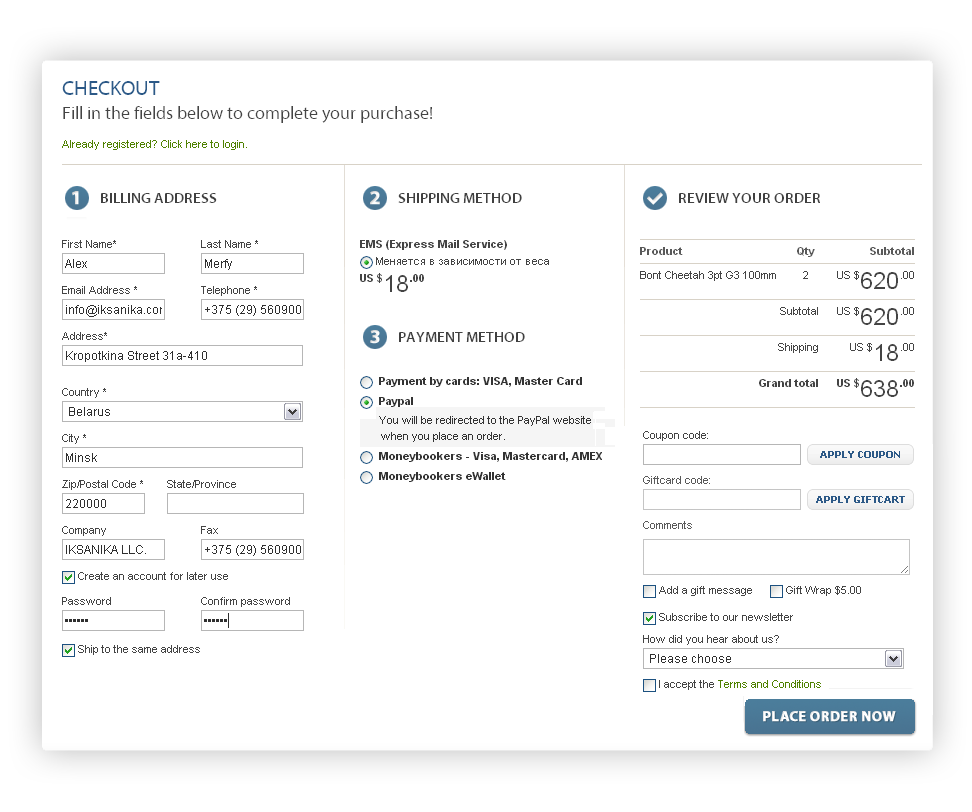The webpage displayed is a checkout screen for an e-commerce platform featuring a straightforward and minimalistic layout, characterized by three primary columns. 

At the top, "Checkout" is written in a light blue font, accompanied by instructions to fill in the required fields to complete the purchase.

**Column One: Billing Address**
- A blue circle with the number "1" indicates the billing address section.
- The form fields for the billing address are: First Name, Last Name, Email Address, Telephone, Address, Country, City, Zip/Postal Code, State/Province, Company, and Fax.
- There is an option to create an account for future use, which includes fields to set and confirm a password.
- The fields are pre-filled, showing an individual from Minsk, Belarus.

**Column Two: Shipping and Payment Methods**
- Step 2, denoted by a "2" inside a circle, covers the "Shipping Method".
  - The selected shipping method is described in Cyrillic.
  - The shipping cost is displayed as USD $18.
- Step 3, part of the same column, pertains to "Payment Method".
  - The chosen payment method is PayPal.

**Column Three: Order Review**
- Topped with a blue circle containing a tick mark, this section is labeled "Review Your Order".
  - The customer has chosen to purchase two units of a product called "Bont Cheetah 3.G3 100mm".
  - The subtotal for the items is USD $620.
  - Adding the shipping fee of USD $18, the total amount is USD $638.
- There are fields for coupons, which remain unused.
- An option to subscribe to the newsletter is available via a checkbox.
- At the bottom right corner, the "Place Order Now" button is prominently displayed.

The design is clean, functional, and ensures users can navigate through the checkout process efficiently.